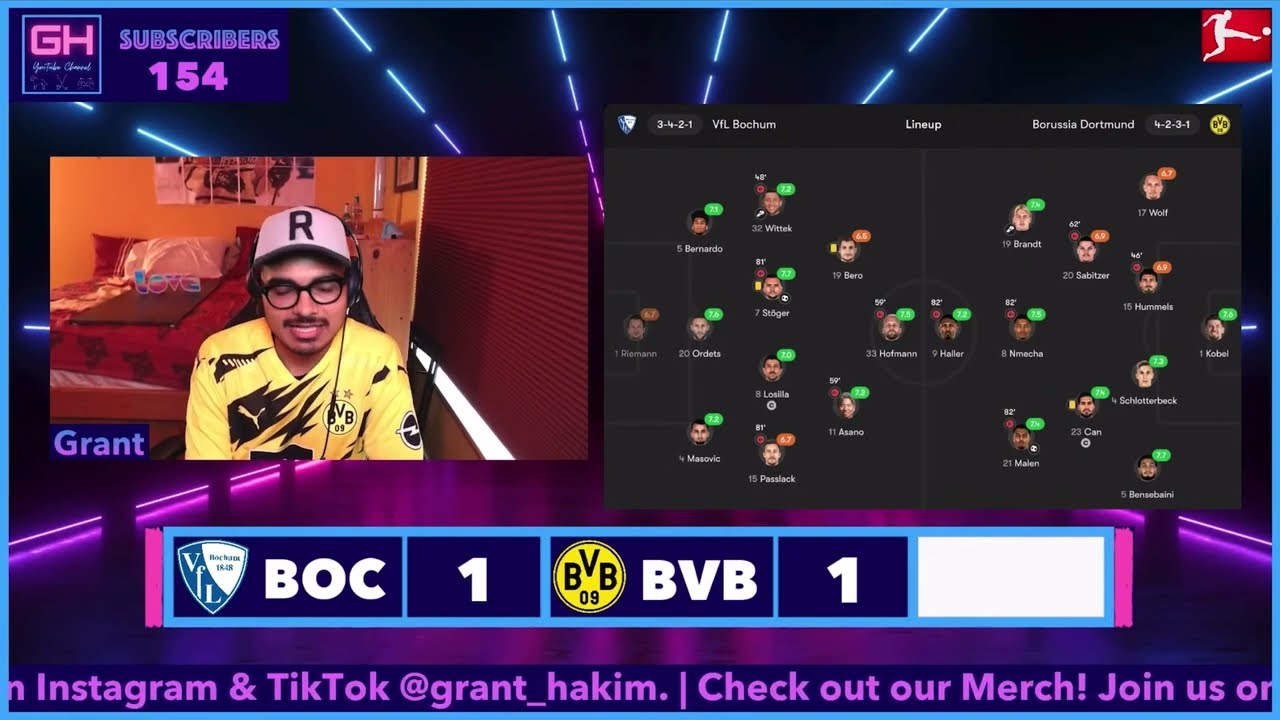The image depicts a screenshot of a Twitch or TikTok stream featuring a man who appears to be an African-American or Latino gamer. He is wearing a yellow t-shirt emblazoned with a black lightning bolt and a yellow Puma logo. He also dons a white baseball cap with a prominent capital "R" on it, black glasses, and headphones with a visible cord. His mustache and goatee are black. The streamer is sitting at a computer desk, likely in his bedroom, as a bed with the word "love" written across it is visible in the background. The room is dimly lit, with burgundy-colored shades drawn down over a window.

In the upper left corner of the screen, there is a pink square with the initials "GH" and a text indicating "subscribers 154." Below the streamer’s image, which is positioned to the left, is a scoreboard displaying "BOC 1" and "BVB 1." A scrolling text at the very bottom announces "Instagram and TikTok at Grant_Hakeem" alongside "check out our merch," although the latter part is partially cut off. 

The background of the game screen features a dark, Tron-like aesthetic with white or bluish rays radiating from the ceiling. On the right side of the image, there are multiple portraits of individuals with different colored message boxes and numbers next to their heads, forming what looks like two team lineups. In the center-right portion, there is a black section with text at the top, and various heads with green or brown message boxes emanating from them. The user's handle, "Grant Hakeem," is displayed prominently in the lower-left corner of the image.